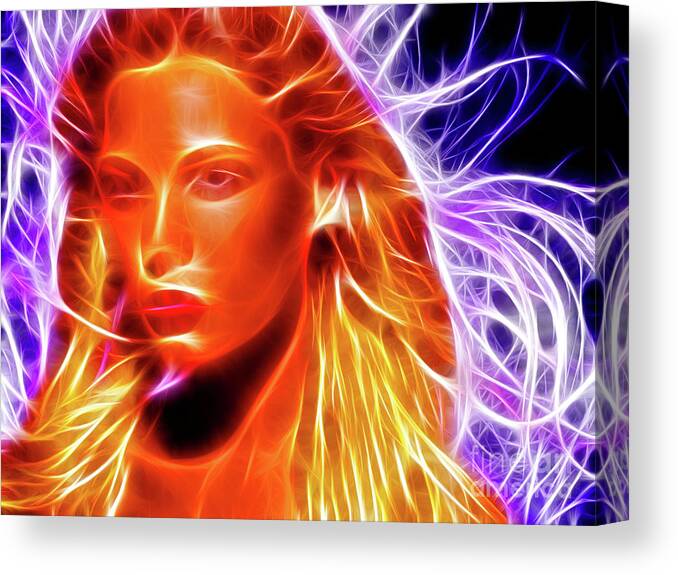This image features a striking graphic art print of a woman with long hair depicted in vibrant shades of orange, yellow, and red. Her hair transitions through various hues, including white, purple, and blue, creating a dynamic and flowing effect that resembles electricity or flames. The woman's expressionless face is turned forward, seemingly gazing out of the frame. The background is predominantly black with intertwining lines of purple, white, and blue that give the impression of energetic currents or waves of electricity.

The artwork appears to be computer-generated and has a noticeable 3D effect, suggesting it may be a custom-made, framed portrait. It extends to the edges, emphasizing its dimensional quality, as if it could be hung up as a piece of decor. Subtle text is located in the bottom right corner, partially obscured by the fiery elements, and possibly includes the word "America." Overall, this electrifying and vividly colored piece combines elements of digital artistry with a physical, painted presentation.